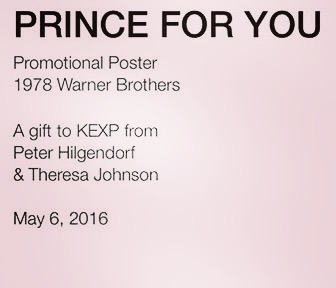The image features a slightly wider than tall, square-shaped promotional poster set against a pale pink background with a subtle gradient, transitioning from almost white at the center to a darker pink at the edges. The top of the poster features bold, all-caps black text that reads "PRINCE FOR YOU," stretching nearly from the left to the right edge of the image. Below, in smaller, left-aligned black text, it says "Promotional Poster 1978 Warner Brothers." Following that, another line reads, "A gift to KEXP from Peter Hilgendorf and Teresa Johnson," and at the bottom, the date "May 16, 2016" is displayed. The overall layout is simple yet elegant, with ample space on the right side of the image, emphasizing the clean, concise text presentation.